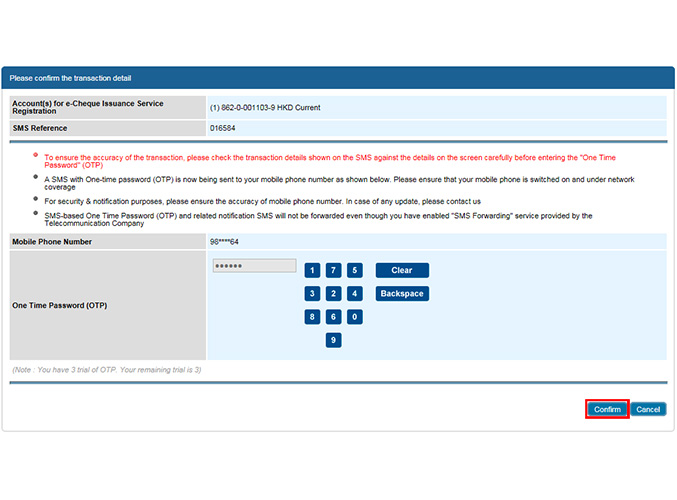This image is a detailed screenshot from an unknown website, depicting a confirmation screen for an e-check issuance service registration. At the very top, the header reads, "Please confirm the transaction detail." Below, it provides account details labeled as, "Accounts for e-check issuance service registration," followed by the account number in parentheses (862-0-001, 103-9), and mentions the currency as "HKD current."

A notification prompts the user to verify the transaction details presented on the screen against those received via SMS. It emphasizes the importance of accuracy before entering a one-time password (OTP). The message informs the user that an OTP is being sent to their mobile phone, urging them to ensure their mobile is on and within network coverage for successful reception. It advises users to verify the accuracy of their mobile number and to update it if necessary by contacting the service provider. An important security note states that SMS-based OTP and related notifications will not be forwarded, even if the SMS forwarding service by the telecommunication company is enabled.

In the screenshot, the partially obscured mobile phone number is displayed as 96****64. Below it, an OTP input box is visible, where the entered OTP is masked for privacy with black circles. Adjacent to the input box, a phone-style keypad with a somewhat unusual layout is displayed, arranged in the following sequence from top to bottom: 1-7-5, 3-2-4, 8-6-0, and 9. To the right of the keypad, there are "clear" and "backspace" options.

A note below the input area states, "You have three trial of OTP. The remaining trial is three." At the bottom of the screen are two blue rectangular buttons labeled "Confirm" and "Cancel." The "Confirm" button is highlighted with a red rectangle, indicating that it is selected.